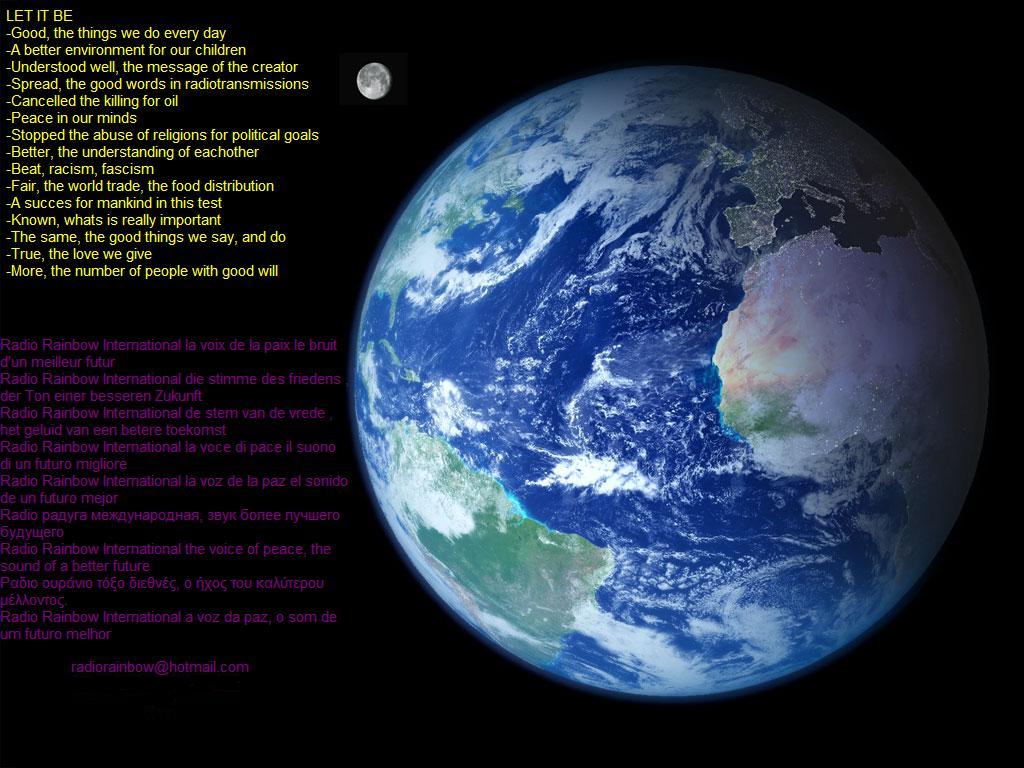The image depicts a vast space scene with the Earth prominently centered against a black backdrop, its blue hues sharply contrasting with the dark void. To the upper left of the Earth, the distant Moon is visible. On the left side of the image, set in yellow text at the top, the phrase "Let it be" stands out, followed by an extensive message advocating for various global and humanitarian improvements. This text reads: "Good the things we do every day, a better environment for our children, understood well the message of the creator, spread the good words in radio transmissions, cancel the killing for oil, peace in our minds, stop the abuse of religions for political goals, better the understanding of each other, beat racism and fascism, fair the world trade, the food distribution, a success for mankind is the test, known what is really important, the same the good things we say and do, true the love we give, more the number of people with goodwill." Below this yellow text, there is a section written in purple, though the details of this text are illegible and it appears to be in a foreign language, possibly French or Russian. The image as a whole evokes a poetic, perhaps even biblical, appeal for global unity and peace, possibly resembling a poetic postcard or a motivational pamphlet.